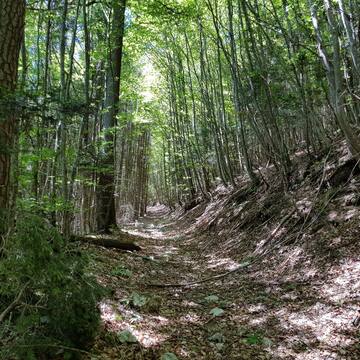This image captures a picturesque forested trail meandering through a serene and inviting woodland. The trail, nestled in a gentle dip, is flanked by an array of slender tree trunks, predominantly a few inches thick, with occasional thicker trunks measuring up to eight or nine inches. These trees form a dense, lush canopy overhead, casting dappled shadows and allowing only patches of sunlight to filter through, illuminating the trail sporadically with bright, natural light. 

The trail is a mix of earth and rocky patches, enhancing the natural aesthetic of the forest. On the left, a noticeable shrub adds to the diversity of the greenery. Despite the ample shade provided by the canopy, glimpses of the blue sky and wisps of white clouds are visible through the leaves, adding a touch of openness to the enclosed pathway. 

This hilly terrain, with trees on either side rising from slight slopes, creates a cool and shaded environment perfect for a refreshing walk or perhaps even a mountain biking adventure on a warm summer day. The overall ambiance of the forest, with its interplay of light and shadow, earthy tones of brown and green, and the natural beauty of its flora, invites tranquility and a sense of escape into nature.